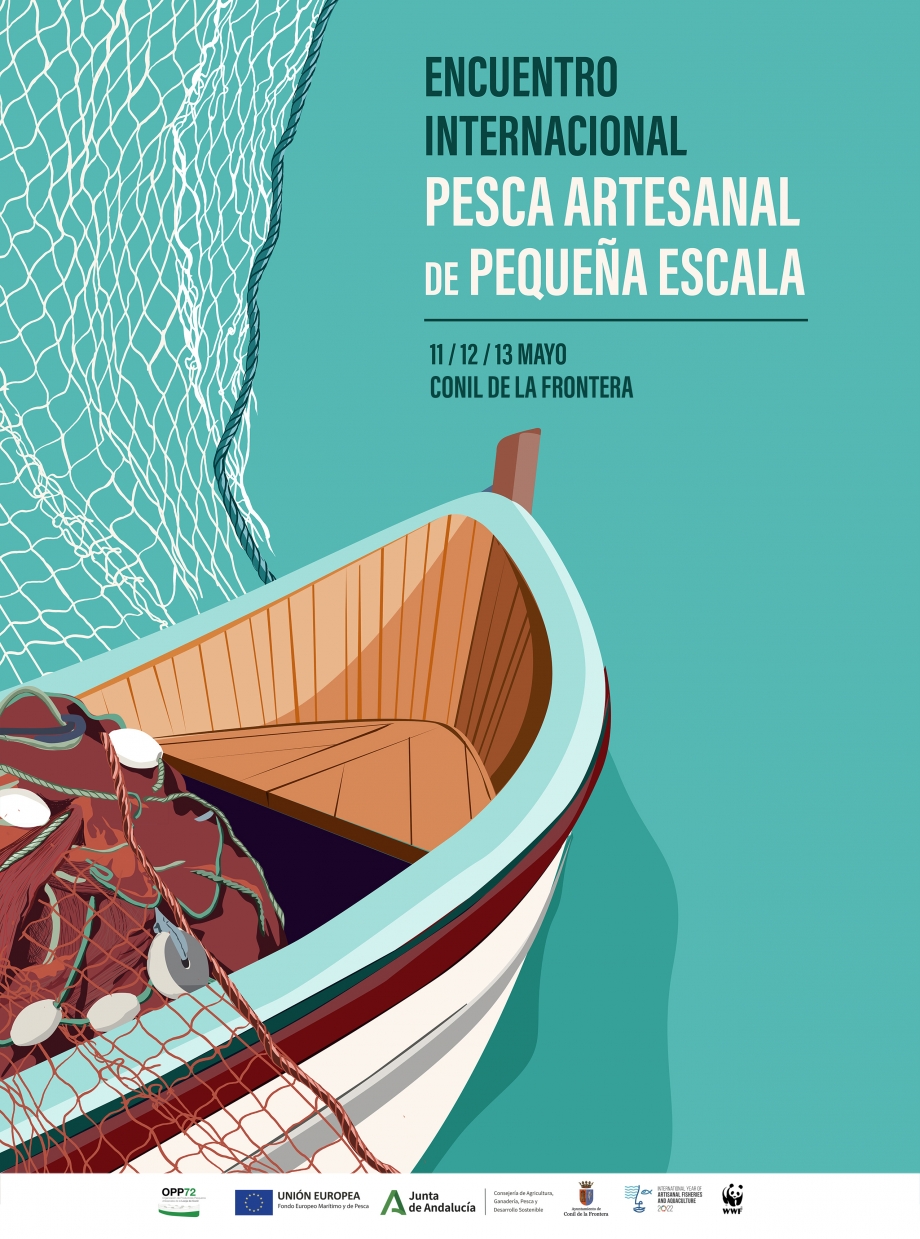This vibrant poster, set against an aqua or turquoise background, announces an event titled "Encuentro Internacional Pesca Artesanal de Pequeña Escala," taking place on May 11-12, 2013, in Conejo de la Frontera. The poster features a detailed illustration of a wooden boat positioned in the lower left corner. The boat has a white-painted bottom hull, accented with a blue streak and a darker red streak below it. Its rim is a light blue, blending harmoniously with the background. The boat contains various fishing nets, including one that is entangled and holds a mass of pale purple objects, and another, differently colored, hanging over the side. The Spanish text, presented in dark blue and white letters, is displayed prominently in the top right corner, adding to the poster's striking design.